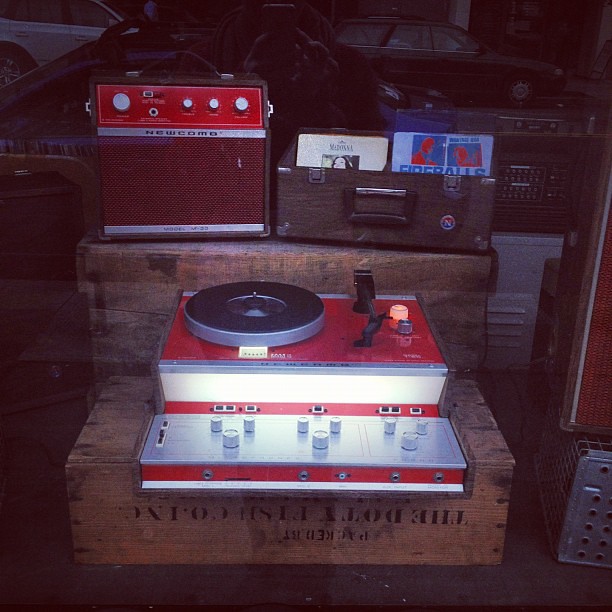The image depicts a vintage DJ setup with a classic turntable system, evoking the style of equipment used in the 1980s. The centerpiece is an aluminium and red metallic turntable deck adorned with a glowing light, various knobs, and headphone sockets. This turntable rests on a wooden step - a two-step structure with the first step displaying some writing on its front kickboard, albeit upside down and partially illegible. The top step houses a matching red and silver subwoofer.

To the right of the subwoofer sits a wooden crate filled with records, including 7-inch singles. An amplifier, possibly bearing the brand name Newcombe, is placed atop this crate. The overall setup is framed against a dimly lit background, where the silhouettes of several cars and additional, indistinguishable hi-fi equipment can be discerned.